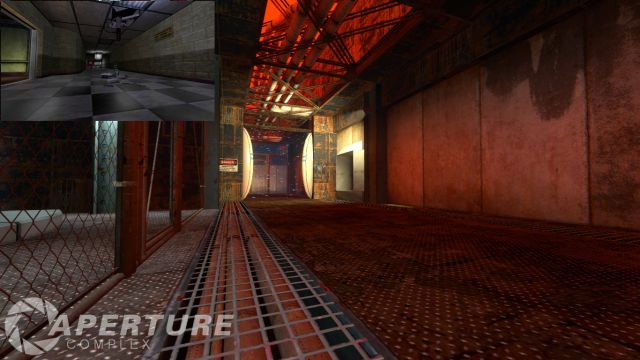The computer-animated image showcases the interior of what appears to be a warehouse or factory, intricately detailed with a metal and industrial aesthetic. The floor is a distinct brownish-orange corrugated steel, with a section on the left featuring a metal grate covering three pipes. The left wall is secured with a gray chain-link fence, while the right wall is composed of gray concrete with an orange tint. Overhead, three metal pipes run along the ceiling's center, emitting a subtle orange glow towards the back. The far end of the hallway reveals two pillars flanking a doorway, with a danger sign posted on the left pillar. Additionally, the top left corner of the image contains a smaller inset picture that depicts a room with a black and gray checkered floor and stone walls. The bottom left corner of the main image bears a watermark reading "Aperture Complex" accompanied by a circular logo.